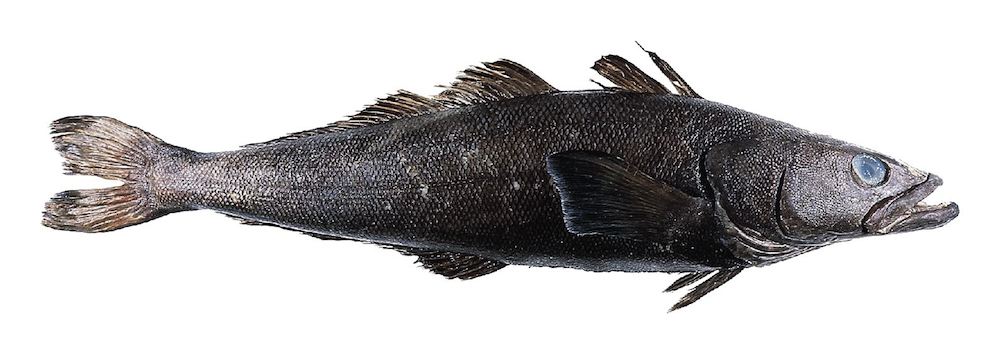The image showcases a dried, scaly fish against a plain white background. The fish, exhibiting a shiny black coloration with some hints of gray and brown, is facing to the right with its mouth slightly agape, revealing a somewhat toothed interior. Its eyes are glassy, indicative of its lifeless state. The fish's body is elongated and intact, bearing all its defining features, including a dorsal fin, a pair of fins past its gills, and a tail with split fins. The dorsal and lower fins appear crusty and dried, with hair-like appendages adorning the top and bottom of the fish, likely aiding in its swimming when it was alive. The overall appearance and attributes, including its scaly texture and fin details, suggest it might be a type of carp, potentially an Asian carp, known for its invasive and aggressive behavior in ecosystems such as the Great Lakes.